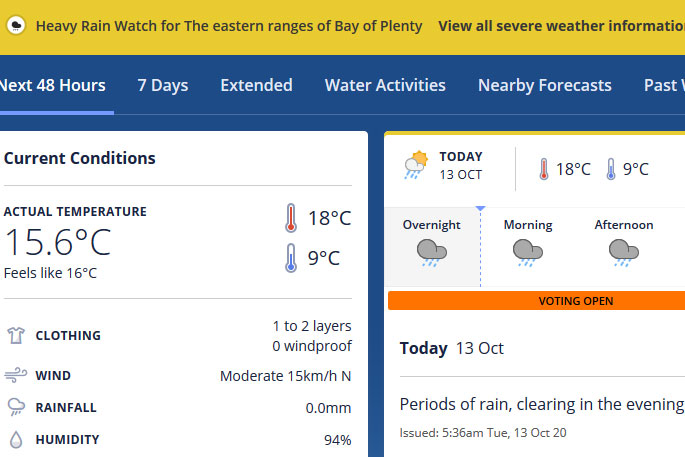The image presents a detailed weather forecast and current atmospheric conditions for the Bay of Plenty area. The top portion of the image features a yellow rectangle with a white circle, presumably an alert icon, which contains black text reading, "Heavy Rain Watch for Eastern Ranges of Bay of Plenty." Below, a slightly cut-off message prompts viewers to "View all severe weather information."

A blue rectangle underneath contains text in white that reads "Next 48 Hours," accompanied by a blue underline. Following this, it lists "Seven Days Extended," "Water Activities," "Nearby Forecast," and "Past," with the latter part of the text partially cut off. 

In the center, there is a white box labeled "Current Conditions," sectioned by a thin gray line. It details the actual temperature as 15.6°C, with a "Feels Like" temperature of 16°C. The box also displays two thermometers: the red one indicating 18°C and the blue one showing 9°C. 

Additional details under the white box include icons for clothing, wind, rainfall, and humidity, each with respective descriptors to the right.

The right-hand side of the image features a smaller yellow bar at the top, below which is an icon displaying a sun, a cloud, and raindrops, labeled "Today, 13 OCT." A vertical line divides this section, displaying a red thermometer indicating 18°C and a blue thermometer marking 19°C. It provides forecasts for "Overnight," "Morning," and "Afternoon," each accompanied by icons of a cloud with rain. 

An orange rectangle highlights that "Voting Open," situated just above another date reminder, "Today, 13 OCT." Below this, a gray line introduces the forecast: "Periods of rain, clearing in the evening," accompanied by the issuance time, "5:36 AM, TUE, 13 OCT 20."